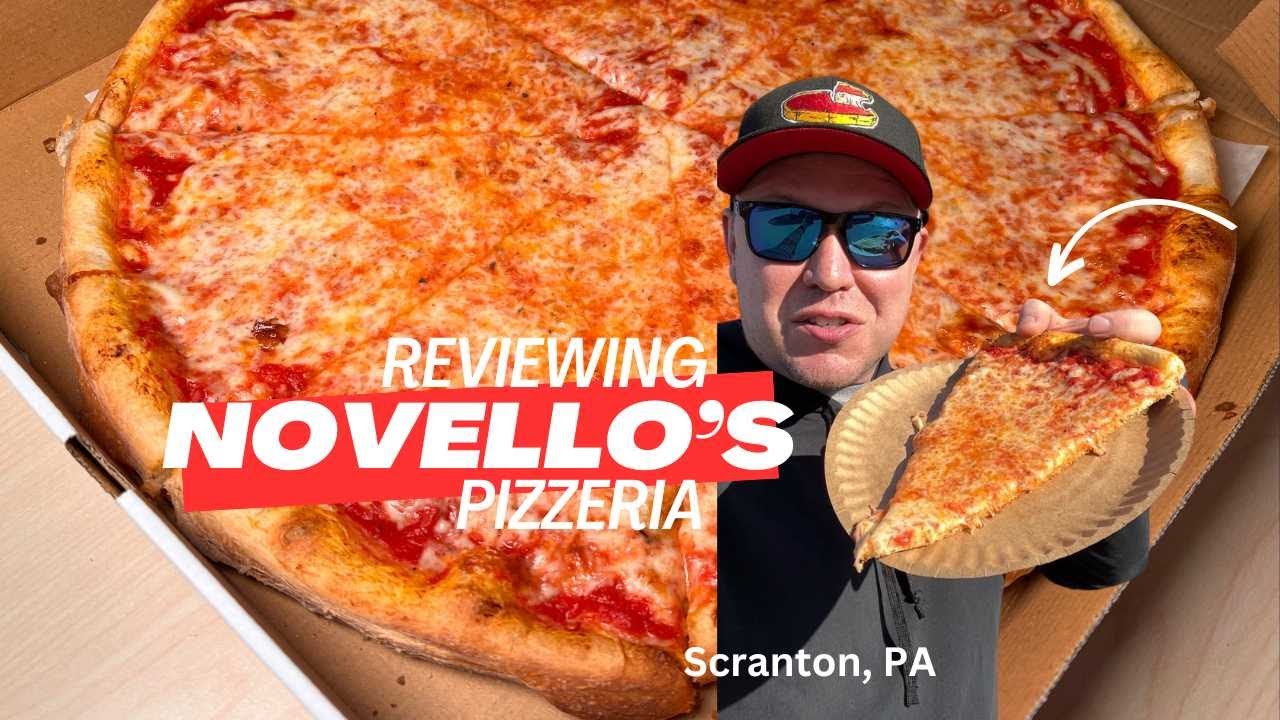This image appears to be an advertisement for Nobello's Pizzeria, prominently featuring a tantalizing, large cheese pizza that occupies about 80% of the visual space. The golden, bubbling cheese topping the pizza looks fresh and delicious, sitting invitingly in a typical cardboard pizza box atop a sheet of wax paper.

In bold, blocky text within the image, the message "Reviewing Nobello's Pizzeria" is visible, with "Nobello's" set against a cockeyed, reddish-colored box backdrop for emphasis. 

To the right of the message, there is a photograph of a man who adds a personal touch to the advertisement. He appears to be casually dressed in a black shirt with "Scranton, Pennsylvania" printed across it, indicating the pizzeria's location. He wears a black hat with a pizza motif, likely representing Nobello's Pizzeria, and accessorizes with stylish black-framed, blue-tinted sunglasses. He is smiling and holding a slice of the appetizing pizza on a brown paper plate, seemingly ready to take a bite.

The overall image is a well-composed advertisement, effectively showcasing the mouthwatering appeal of Nobello's Pizzeria's cheese pizza while highlighting its local roots in Scranton, Pennsylvania.